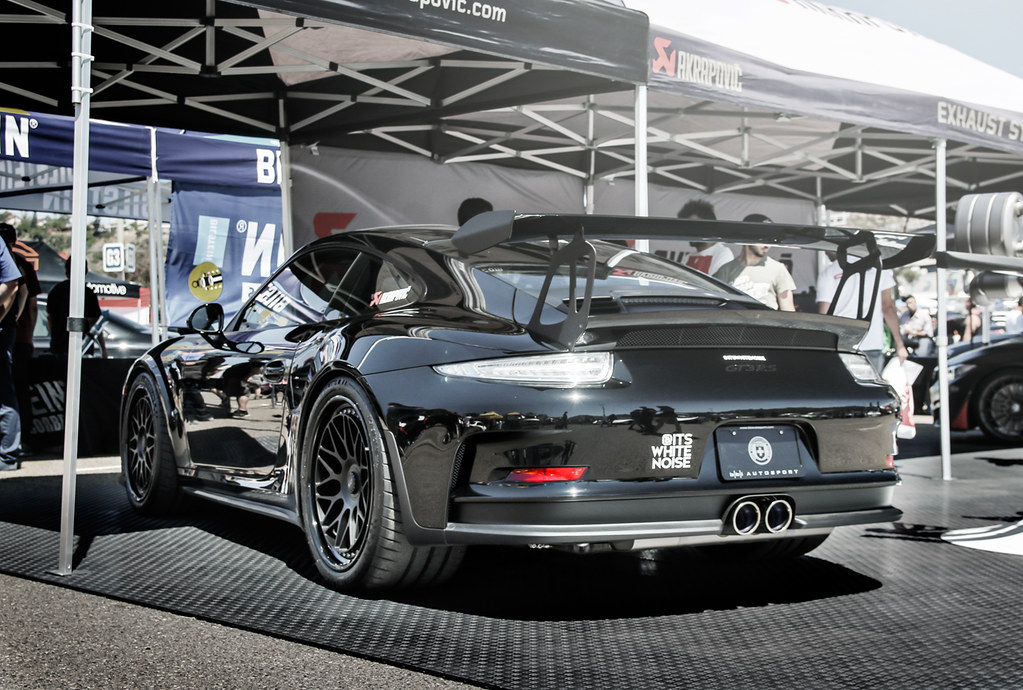The image depicts the rear view of a black Porsche 911 GT3 RS, a high-performance sports car, on display at an outdoor racing event. The car is parked on a black rubber mat and is partially sheltered under a white tent with a metallic framework, shielding the front half while the back protrudes into the sunlight. Advertisements for tires and high-performance exhaust systems, including the brand "AKRAPOVIČ," adorn the tent sides in white print on black fabric.

The car's rear features distinctive elements like a prominent spoiler and dual exhausts centered above the bumper. The shiny, polished surface of the car is highly reflective, capturing the image of the photographer and the spectators in the background. A humorous bumper sticker reading "It's white noise" is affixed above the area where the license plate would be. The surrounding environment includes several other vehicles in the distance and numerous spectators, predominantly men, casually observing the display. The scene is set on a sunny day, enhancing the visual appeal of the car and adding a vibrant atmosphere to the racing event.